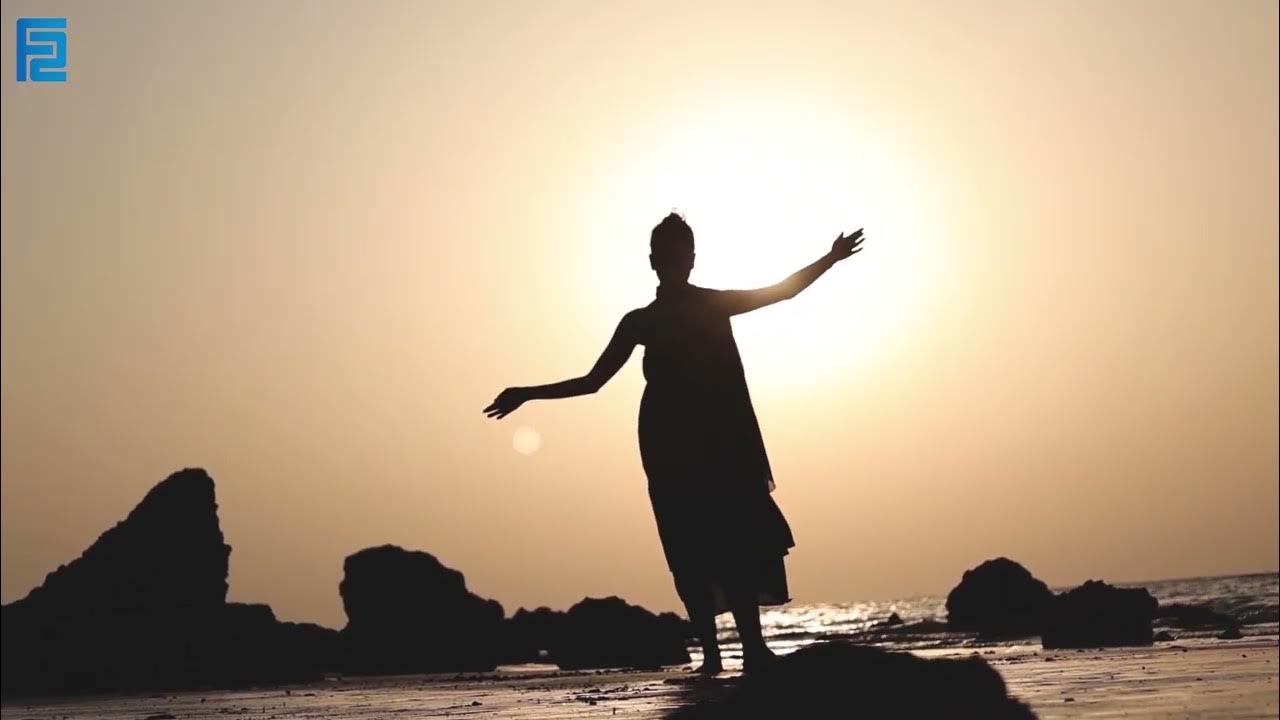The image depicts a silhouetted figure standing on a beach with their arms outstretched, facing the sun. The person appears to be female, dressed in a long, sleeveless robe or dress, with hair likely tied up in a bun, although specific details are obscured by the silhouette. Their form is stark black against the backdrop of a striking sky, transitioning from a bright, radiant sun at the center to a golden-tan and orange gradient extending outward. The sand beneath their feet is wet, reflecting the light, while jagged rocks protrude around them, partially obscuring their feet. The ocean reflects the low sun, creating a small orb of light below the person's left hand, adding a mystical touch to the scene. In the upper corner of the image, a blue logo with an interlocking uppercase "F" and the number "2" is visible.